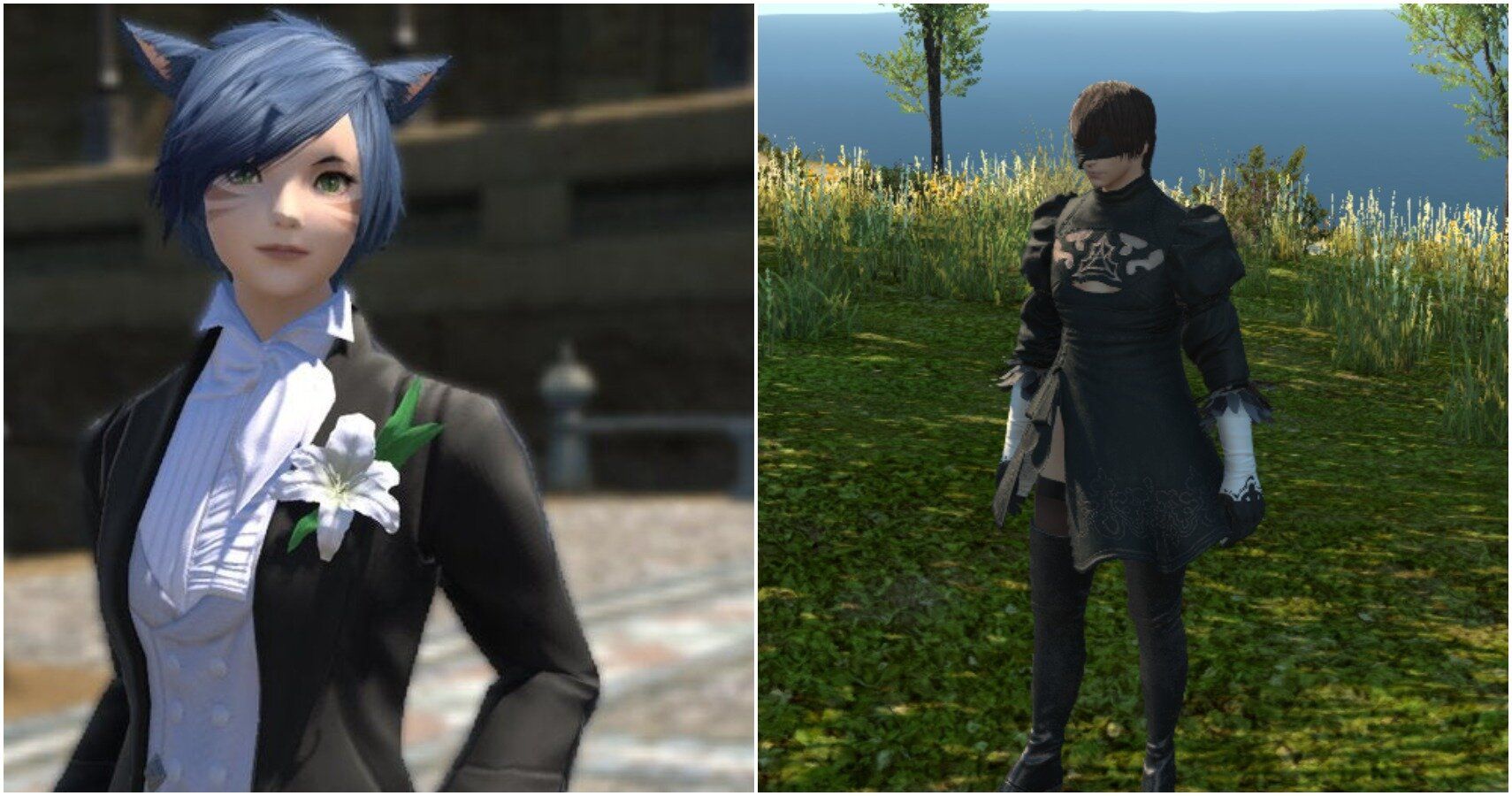The landscape image is divided by a white border into two square images. The left square showcases a digitally created character resembling a young woman, who has short, blue, emo-style hair with triangular cat ears. Her face, which features painted whisker-like stripes on the cheeks, appears human with fair skin and green eyes. She is dressed in a sophisticated outfit comprising a button-down shirt, a blue double-breasted vest, a black suit coat adorned with a large white, green, and yellow flower on the lapel, and the background is partially blurry with black at the top and tan or gray at the bottom.

The right square highlights another detailed 3D character, a young man blindfolded with a black cloth that drapes unevenly across his face. His attire is a black Victorian-style ensemble with tight black pants, a long-sleeve dress featuring puffy shoulders and white lacy cuffs that meet at his forearm, a large slit revealing his upper thighs, and tall black boots. The background of this character depicts a scenic area with tall grass, small trees, a drop-off cliff, and a large body of water, suggesting it’s late in the day as the sun appears low in the sky. Both animated figures seem to inhabit a video game or Metaverse-like environment.